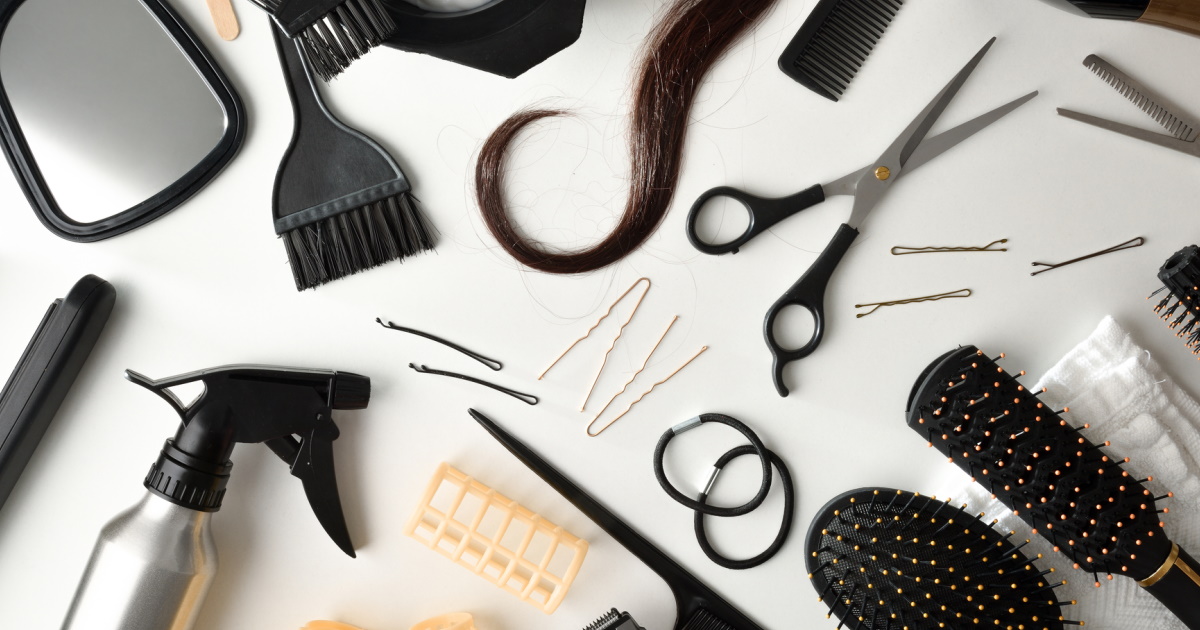This photo, set against an all-white background, displays an aesthetically arranged collection of hairstyling tools, meticulously laid out as if in a hairdresser's salon. Prominently featured is a handheld mirror with black trimming, positioned in the top left, angled toward the bottom right. A metallic-bottomed spray bottle sits in the bottom left, angled upward. Nestled amidst these items is a brush used for applying hair dye, positioned diagonally. Noticeably, a pair of open scissors lies slightly to the middle right, pointing toward the top right. Scattered throughout the image are various bobby pins, both traditional and larger gold ones, strewn in different directions. 

Additionally, the layout includes multiple types of hairbrushes: one round, one square, and another unmentioned shape, all situated in the bottom right and angling toward the top left. Here too are ponytail holders and two hair curlers. The photo captures the ends of a comb and the tips of someone's curled hair, adding a layer of realism. A smaller pair of scissors, typically used for layering, is also visible among the items, emphasizing the professional vibe of the display. The overall diagonal arrangement of the tools lends an organized yet dynamic aesthetic to the composition, highlighting essential hairstyling instruments.